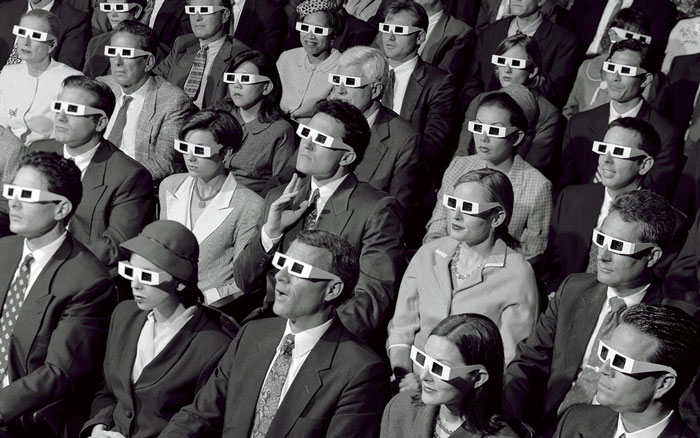A detailed black-and-white photograph captures a scene from a 1950s-style movie theater. The image, in landscape orientation, features multiple rows of men and women dressed in formal business attire – suits, ties, and dresses. Each viewer is seated side-by-side, wearing basic white paper 3D glasses with black rectangles for lenses. The audience, which spans about five rows with roughly five people per row, gazes upward and to the left at a screen outside the frame. The expressions across the crowd vary from smiles to looks of awe. Notably, a man in the middle of the scene lifts his hand under his chin. The photograph showcases a moment of shared experience and excitement in a 3D movie auditorium.